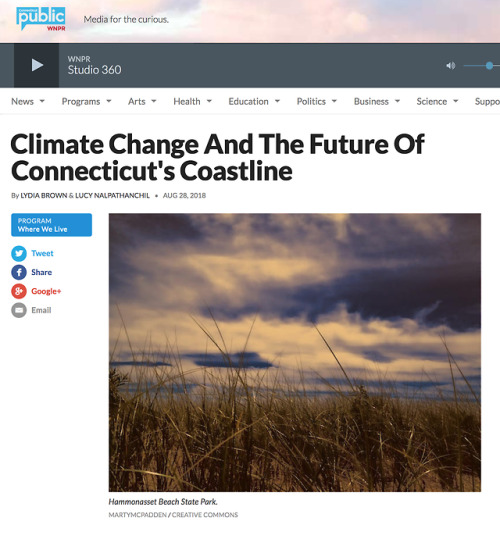Screenshot of the "Public" Website Homepage

The screenshot captures the homepage of a website called "Public," designed for the curious. Central to the image, a play button is prominently displayed, labeled "Studio 360," likely indicating content from WNPR. Above this, navigation elements include a play button and volume icon positioned at the far right of a control bar.

Directly beneath this are various expandable categories marked by upside-down triangles, signifying an array of sections including News, Arts, Health, Education, Politics, Business, Science, and Support. These categorically organized sections aim to provide users with easy access to content based on their interests.

The featured article at the top of the page is titled "Climate Change and the Future of Connecticut's Coastline" by Linda Brown and Lucy, dated August 28, 2018. Below this primary article, a highlighted section titled "Where We Live" appears in a blue box, hinting at a specialized program or series.

In the same area, icons for major social media platforms are displayed, allowing users to share content via Twitter (depicted with the bird logo), Facebook (share icon), Google+ (G+ logo), and email (envelope icon).

To the right side of the screen, the visual focal point is an image of dark, ominous clouds looming over a field of weeds or wheat, labeled as Hammondasset Beach State Park. This backdrop adds a dramatic visual element to the page, enhancing the thematic emphasis on climate and environmental issues.